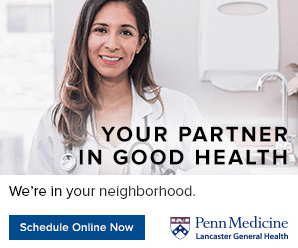**Caption:**

A comprehensive view of the Penn Medicine Lancaster General Health website features a prominent logo reminiscent of a coat of arms. The logo's top segment is red, while an inverted 'V' with blue and white dots is positioned on the bottom right. The bold, black text "Your Partner in Good Health" stands out prominently. Just below, it further reassures visitors with the phrase "We're in your neighborhood," and a call-to-action "Schedule online now" is displayed at the bottom left.

Centrally, there is an image of a woman in the medical profession. She has light skin and brown hair that falls just below her shoulders in a straight style. Her friendly smile is accentuated by a small stud earring visible on one of her ears. She is dressed in a white lab coat with a stethoscope draped around her neck, epitomizing professionalism and care. The background reveals a typical clinical setting, including a box with a paper towel dispenser mounted on the wall and a sink with a faucet on the right, adding authenticity to the healthcare environment.